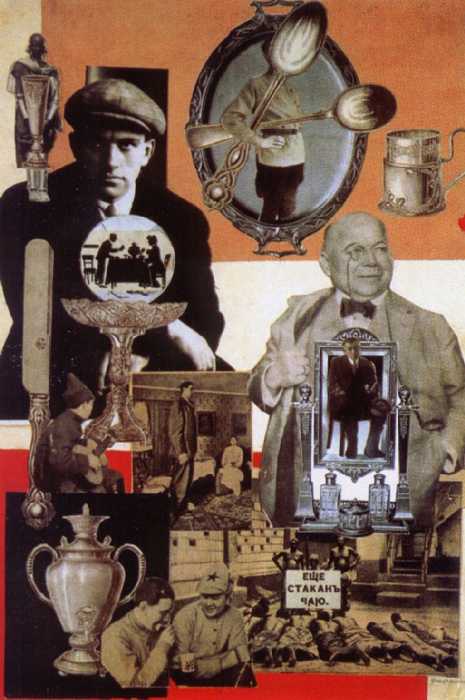The image is a detailed and intricate collage that primarily features two men at its center, wearing distinct attire indicative of the 1940s. One man is in a black suit with a tie, while the other, on the right, sports an old-fashioned eyeglass piece attached to his jacket. The collage includes a variety of objects and people, arranged in a visually engaging manner. Among these are a person holding a gun with spoons tucked in their arms, and another person playing a guitar. There are various household items such as a butter knife on the left, metal dishes, forks, and additional spoons prominently displayed throughout. 

In the top part of the collage, there's a person holding two spoons, and on the left side, a man appears to be staring into the scene. To the right, another individual is holding a picture or a frame. At the bottom, several Soviet soldiers are depicted, suggesting a wartime context possibly linked to the Second World War. The colors in the collage are a mix of red, white, orange, black, and gray, creating a rich visual tapestry.

Within the imagery, there's an inferred presence of Winston Churchill on the right side, which enhances the historical context. The abundance of silverware and the inclusion of military figures suggest a potential critique of wealth accumulation, anti-fascism, or a commentary on communism. The collage seems to evoke themes of conflict, societal commentary, and historical reflection.